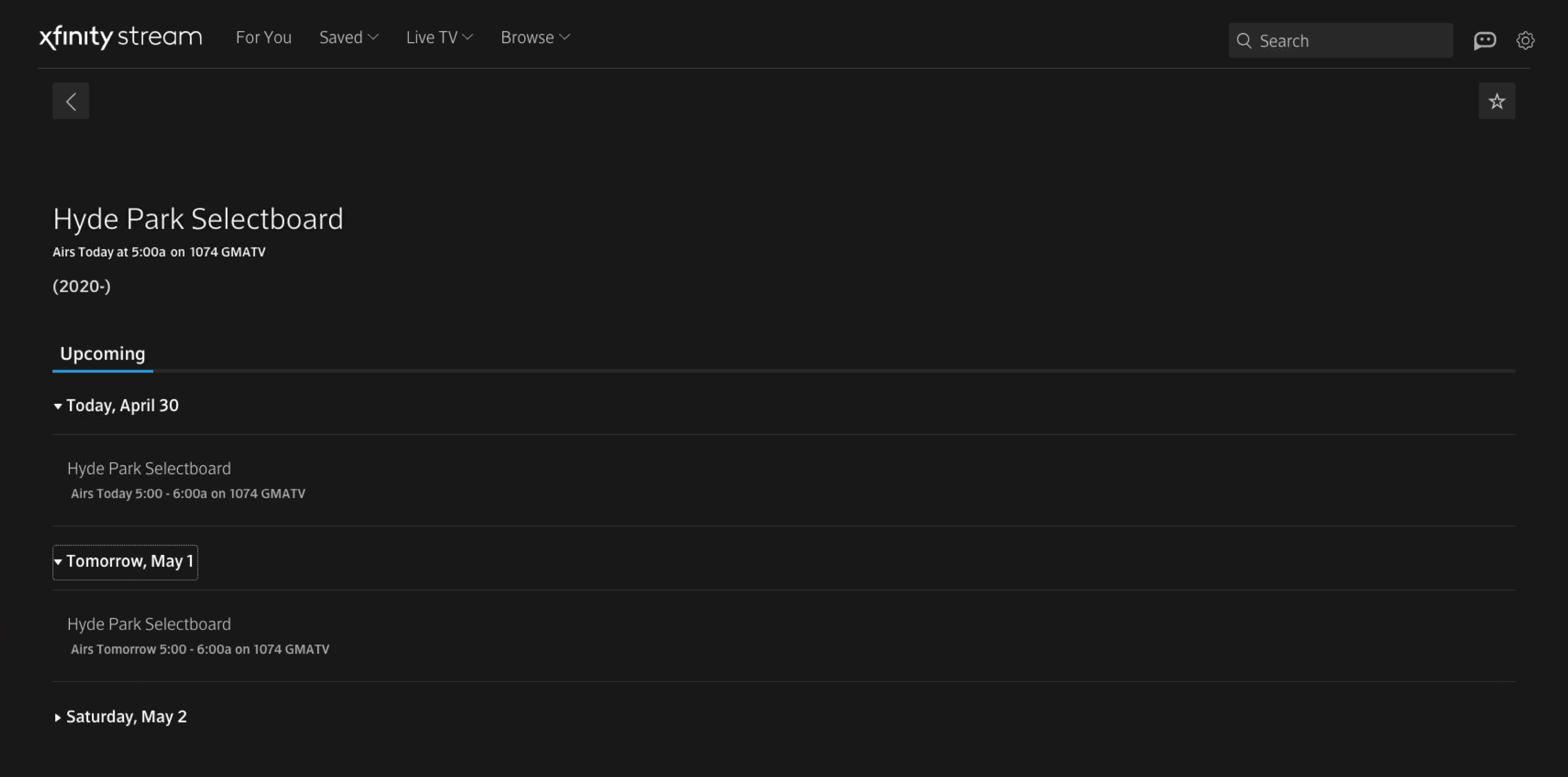The image in question is a screen capture from the Xfinity Stream interface. The layout is rectangular, approximately twice as wide as it is tall, set against a black background. 

At the very top of the image, there is the title "Xfinity Stream" displayed in white text. Adjacent to this title are menu options labeled "For You," "Save," "Live TV," and "Browse," all in gray. On the far right-hand side, there is a search bar.

Beneath the header, on the left side, there is a gray left arrow icon encased in a dark gray square, indicating a back navigation button. On the upper right side, directly opposite the left arrow, there is a white star button also set against a dark gray square. 

Moving further down the left side, large white text aligned to the left reads "Hyde Parked Select Board." Below this, in much smaller white text, it says "Airs Today at 5 a.m. on 1074 GMA TV." Directly underneath, it states "(2020)" with a minus sign in parentheses.

Below these details, there is a menu with only one selectable option labeled "Upcoming," which is underlined in blue to indicate its selection. Under this, the text "Today, April 30th" is displayed in white, accompanied by a down arrow. This section expands into gray text that reads "Hyde Park Selected, Airs Today, 5 to 6 a.m."

The overall design is clean and organized, providing viewers with clear navigation and information about the broadcasting schedule.